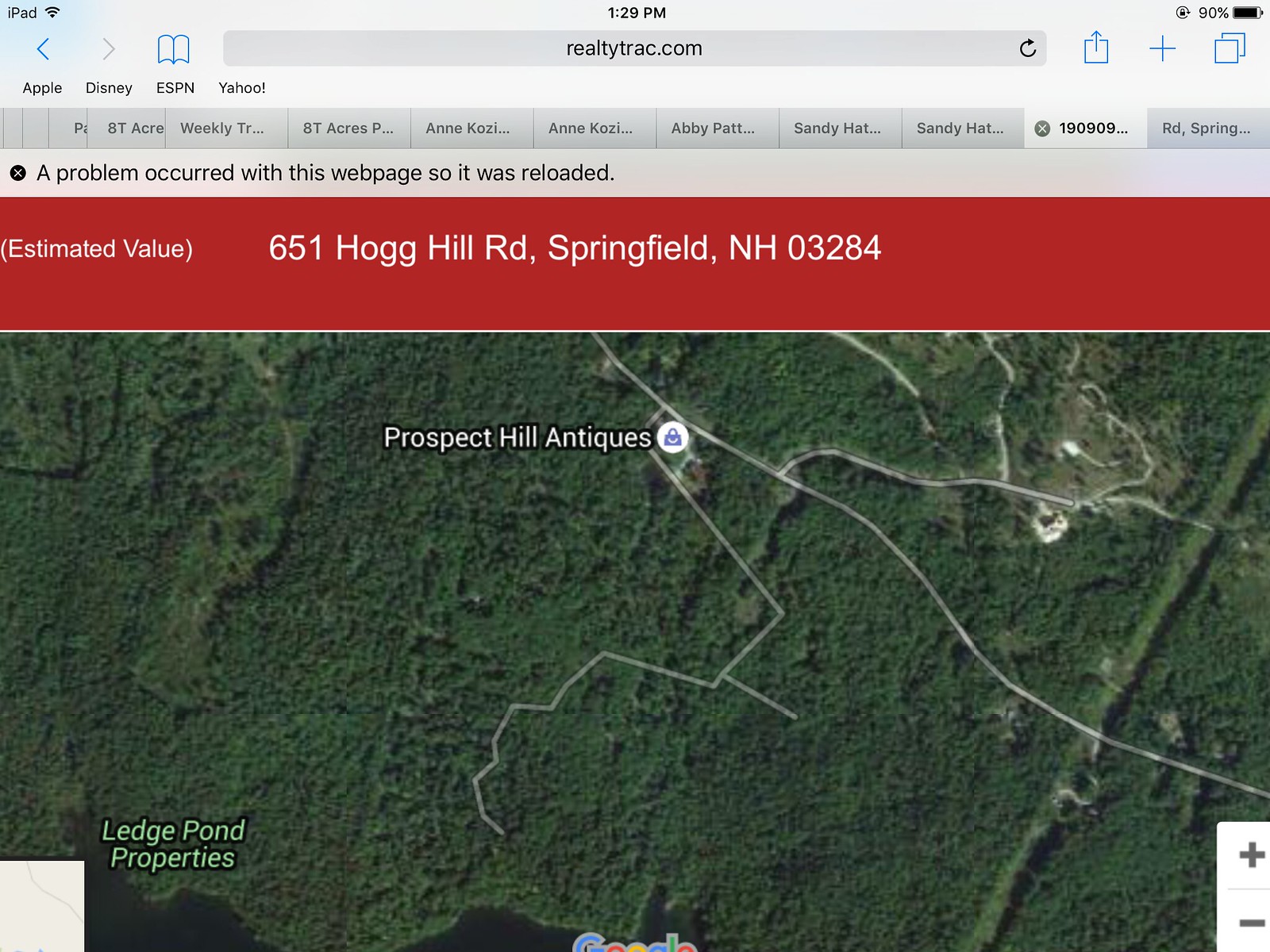The image is a detailed screenshot from an iOS device, likely an iPad, showcasing a website on the Safari browser. At the topmost part of the screen, various typical device icons are visible, including the time, battery percentage, and signal strength. Below these, the address bar displays "RealtyTrack.com," and a secondary gray bar contains multiple icons like Apple, Disney, ESPN, and Yahoo.

A notification in a thin bar states, "A problem occurred with this webpage, so it was reloaded." Following this, a prominent red bar is seen with white text indicating "651 Hog Hill Road, Springfield, NH 03284,” along with the estimated property value.

The primary content occupying the bottom two-thirds of the screen is an aerial map, with notable geographical and property details. The area is lush and green, marked by white lines likely representing roads. Significant landmarks include text reading "Prospect Hill Antiques" to the right of the main address point. At the bottom left, there is additional text in light green, annotating "Ledge Pond Properties.” The map interface includes zoom controls at the bottom right corner and partially visible "Google" text at the bottom middle. 

Overall, the screenshot provides a comprehensive view of a property listing, along with related navigation and annotation features from the real estate website.